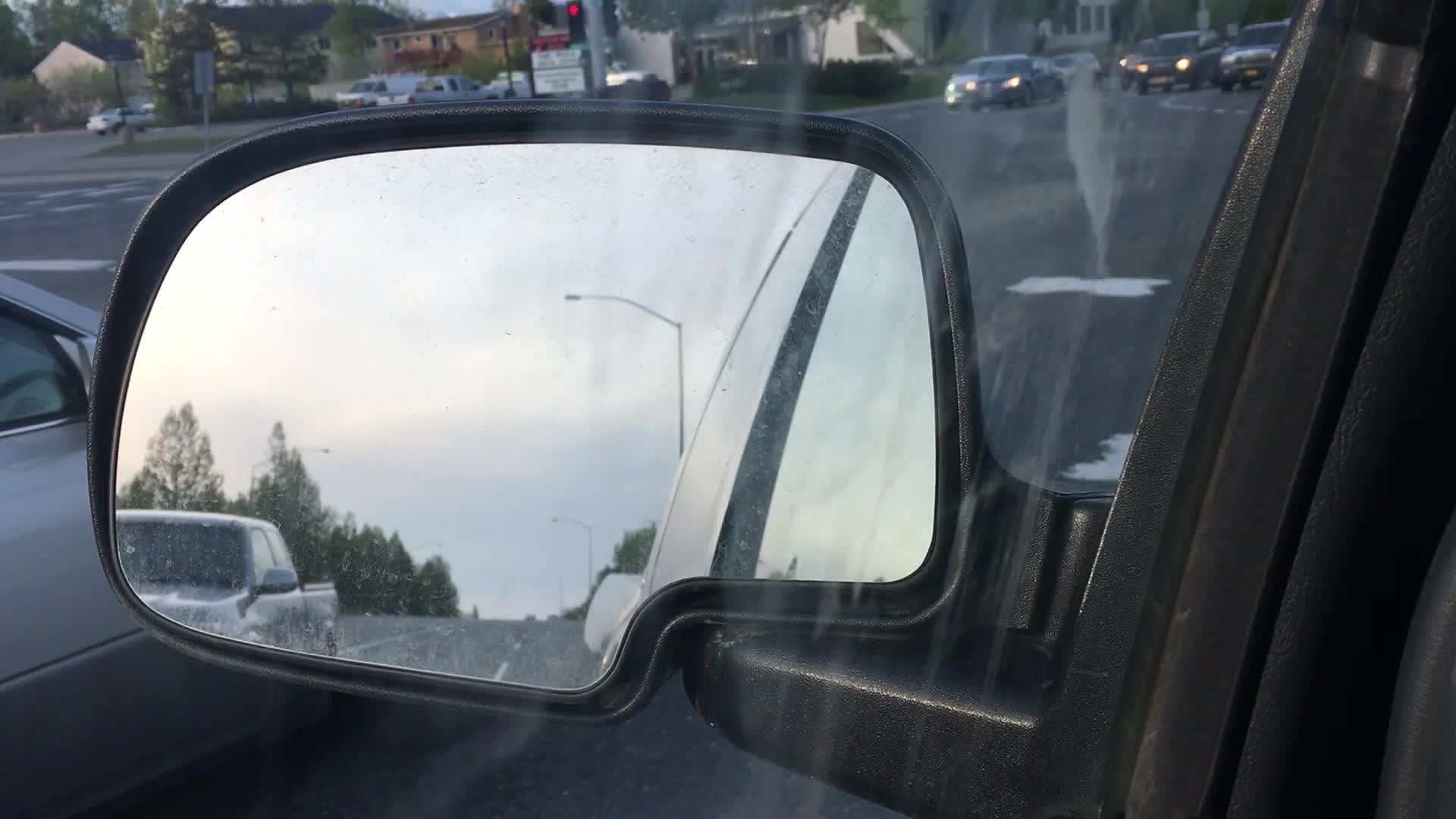A detailed side view from within a vehicle focuses on the left side mirror, capturing a dynamic roadway scene. The mirror, uniquely shaped with a curvature around its supporting arm, reflects a multi-lane road stretching behind. In the reflection, a gray truck advances in one of the adjacent lanes, while a gray car is situated directly beside the viewer's vehicle. The exact color of the vehicle housing the camera remains indiscernible, but the geometry of the mirror adds an intriguing visual element. Beyond the mirror's edge, glimpses of the road reveal several other cars approaching, and in the distance, additional multi-lane traffic is visible, accompanied by residential buildings or similar structures lining the horizon.